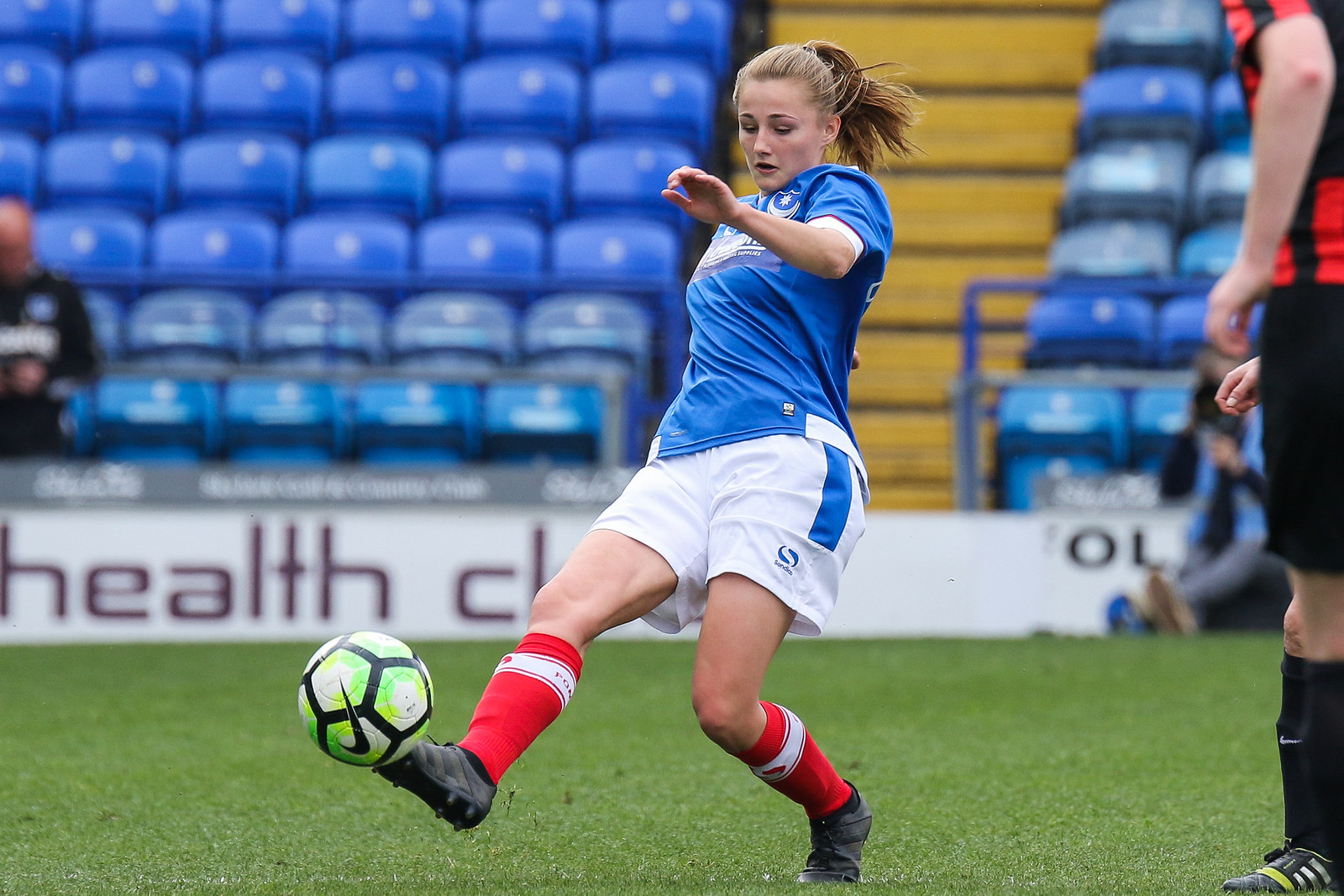In this dynamic sports photograph, a female footballer, with her hair pulled back in a ponytail, is captured at the precise moment she kicks a colorful green, white, and black Nike soccer ball. Dressed in a blue short-sleeved jersey, white shorts featuring a blue stripe, red socks, and black cleats, she displays immense focus and athleticism. Her left foot is firmly planted on what appears to be a carefully maintained, vivid green astroturf field, while her right foot strikes the ball mid-air. The backdrop features an almost empty stadium with rows of blue seats and distinctive yellow steps. To the left, an official in black shorts and a red and black striped jersey stands in observing. The sparse audience includes a blurred figure seated near a white banner, which might belong to a sponsor, possibly a Health Club. A solitary person, perhaps a sports photographer, is positioned in front of the banner, possibly capturing the action from another angle.